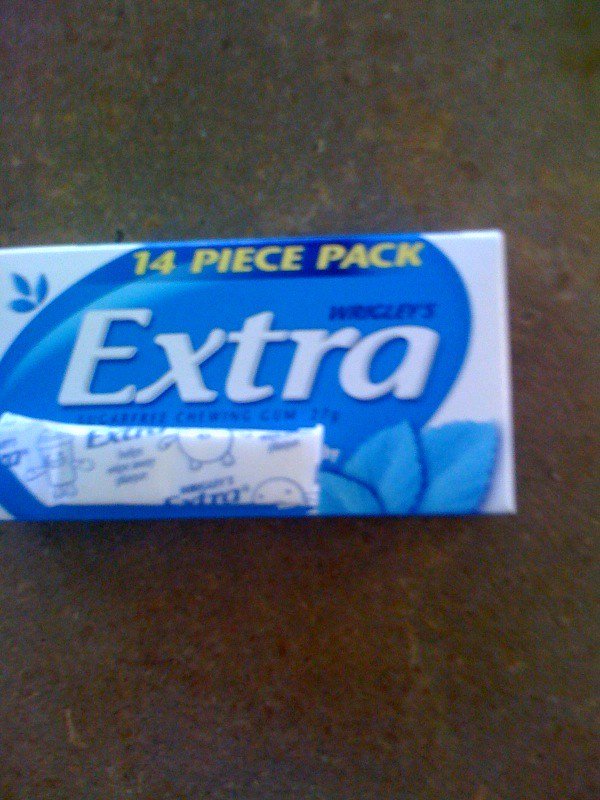This is a close-up image of a 14-piece pack of Wrigley's Extra chewing gum, prominently featuring a mostly blue package with white writing. The package includes a dark blue "Wrigley's" logo and large white "Extra" letters set within a light blue oval on the front. In the bottom right corner of the package, there are subtle illustrations of mint leaves in a lighter blue color. Notably, the words "14-piece pack" are highlighted in yellow on the top of the package. 

A single piece of gum, still wrapped in a mostly white wrapper with blue writing, is placed on top of the pack. The wrapper also features a funny little character. The entire scene is photographed against a mottled marble countertop with predominantly brown tones. The image is notably blurry, making some of the smaller text and details hard to discern.